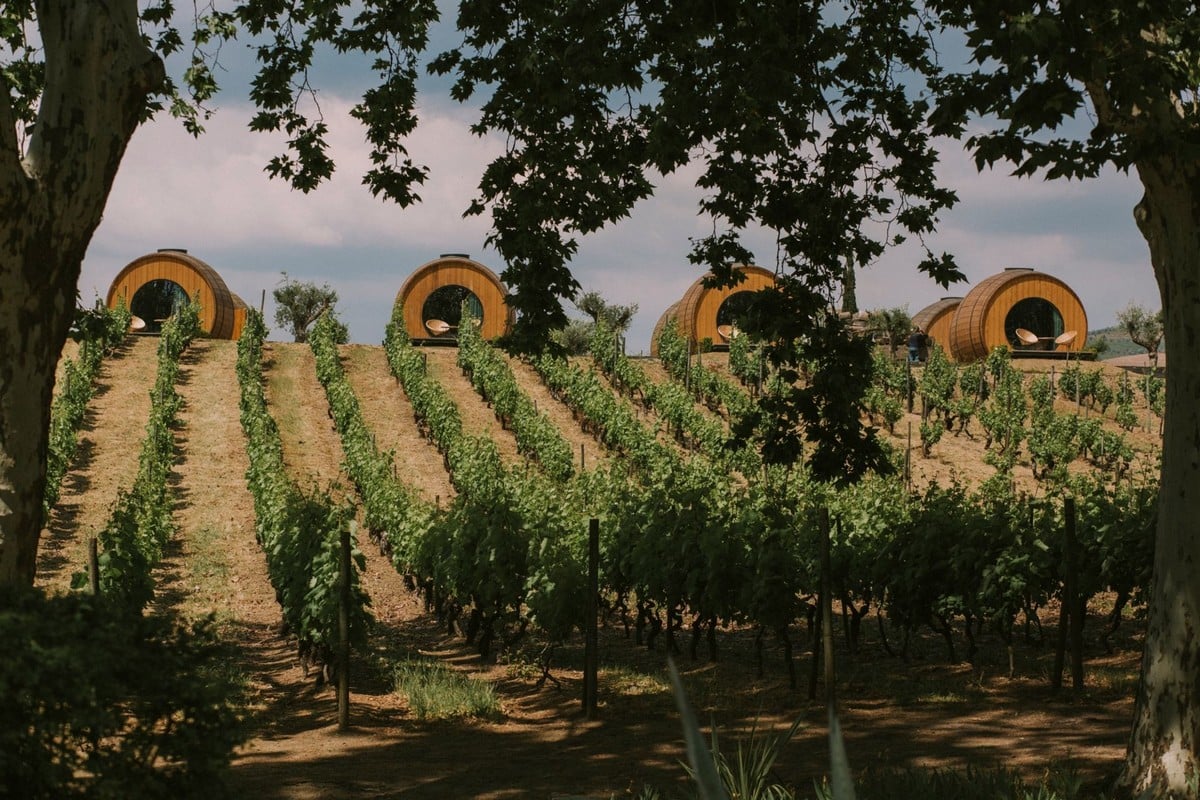This vivid color photograph captures a meticulously cultivated field of crops on a sunny day with clear blue skies peppered with white clouds. In the foreground, the scene is framed by the trunks and overhead branches of two large, leafy trees, casting ample shade over the area. Rows of rich, brown soil alternate with green crops, suggesting an orderly, farmed nature, possibly grapevines supported by trellises, extending towards the horizon. At the top of the hill, there are four striking, large cylindrical structures resembling wooden barrels, adorned in shades of brown, which seem to serve as buildings, possibly storage or seating areas. Each of these barrel-like buildings is accompanied by what looks like a porch with tables and chairs, adding a touch of rustic charm to the idyllic landscape. The absence of people and animals, combined with the high quality of the photograph, highlights the serene, natural beauty of this well-tended agricultural setting.